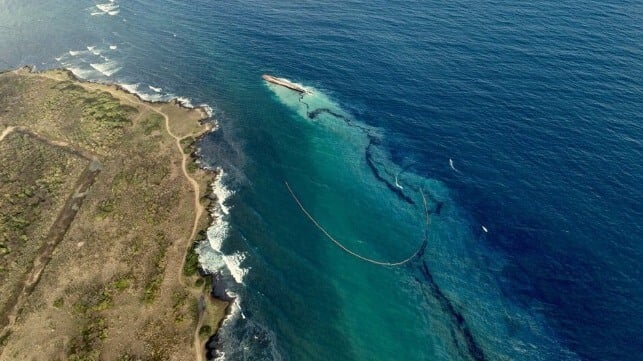This aerial photograph, likely taken from a plane or drone, showcases a dramatic coastal scene. On the left side of the image, a rocky, dirt-covered shoreline with sparse shrubbery juts into a vibrant blue ocean. White waves crash vigorously against the rugged coast. Further out in the water, the blue deepens to a darker hue. Near the center-left, a large, brown object—possibly a boat—is visible, leaving a dark trail behind it which could suggest an oil or gas spill. There's also a distinctive, giant metal hook-like structure partially submerged in the water. Additional smaller boats can be seen further out in the deeper blue waters. This image captures both the natural beauty and the human impact on this striking seascape.